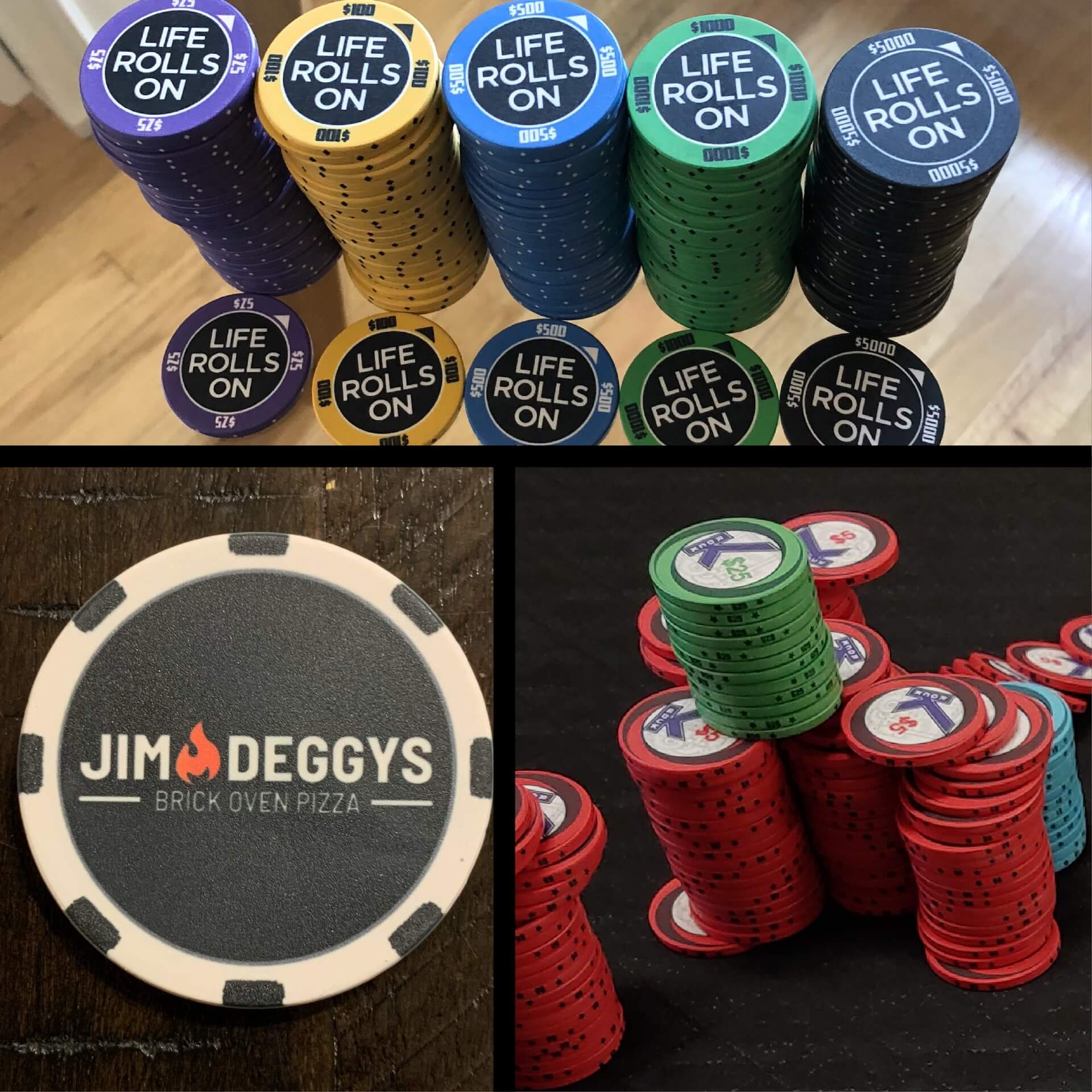This image is a detailed collage consisting of three separate photographs showcasing various sets of poker chips. The topmost rectangular photograph, set against a wooden table, features five neatly arranged stacks of poker chips in vibrant colors: purple, yellow, blue, green, and a dark hue that appears to be either black or dark blue. Each chip prominently displays the text "Life Rolls On" in white block letters centered within a black circle, surrounded by denominations that include $25 on purple, $100 on yellow, $500 on blue, $1,000 on green, and $5,000 on the darkest chips.

Below, the bottom left photograph presents a close-up of a single large poker chip with a dark brown woodgrain background. This chip bears a white outline and edge markings, encircling a black center with white text reading "Jim Deggy's Brick Oven Pizza," accompanied by a red flame graphic following the name Jim.

The bottom right photograph reveals a somewhat haphazard arrangement of poker chips. Predominantly red, the stacks also feature one shorter stack of blue chips and an additional stack of green chips perched atop the red ones. Visible chip denominations range from $5 to $25.